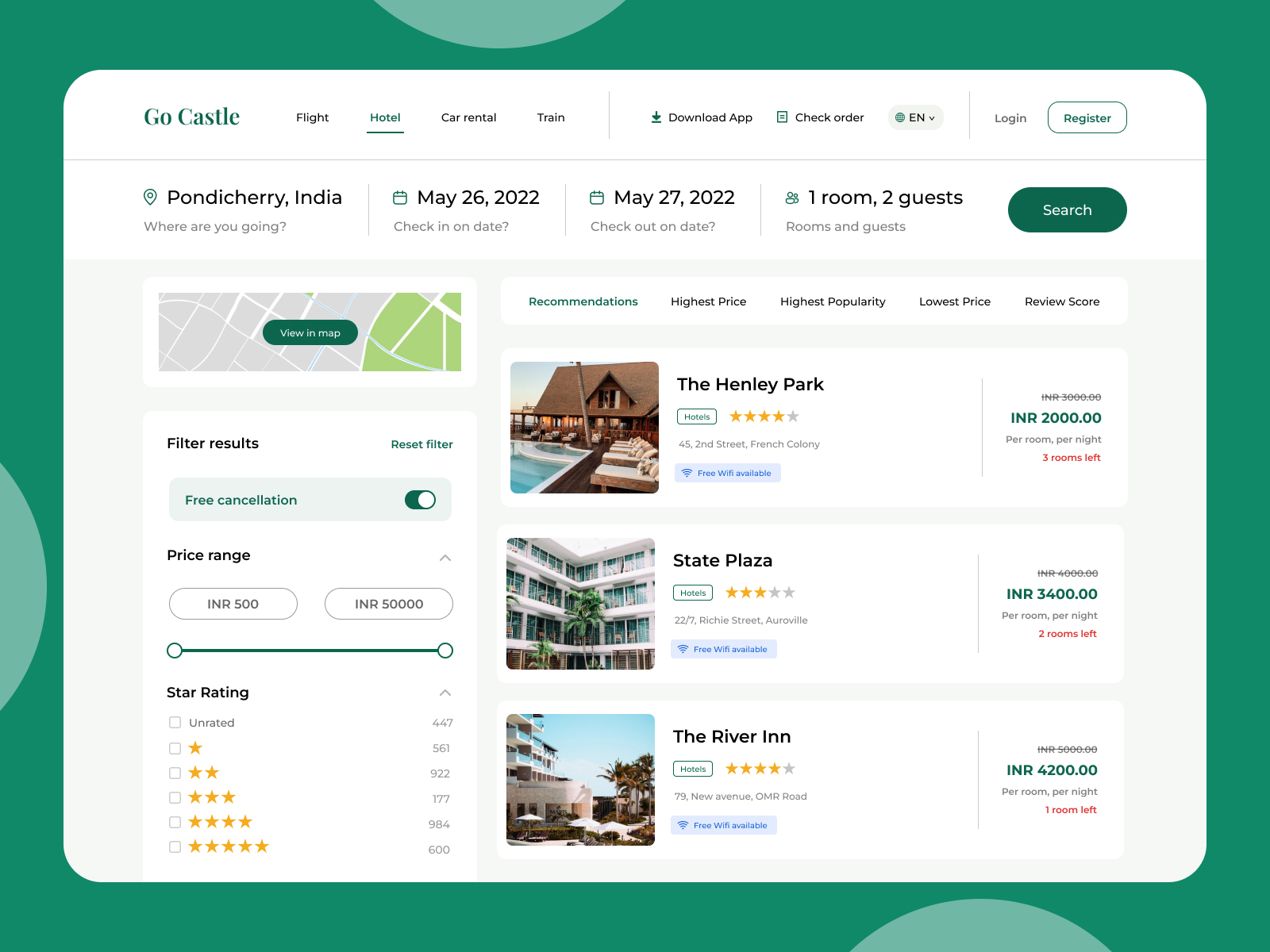The image features a detailed travel booking interface on a green background that appears to form the beginning of a circular design. The interface is divided into distinct sections:

1. **Tabs and Navigation**:
    - On the upper left-hand corner, there are tabs labeled "Gold Castle" in green, "Flight" in black, "Hotel" in green (underlined, indicating the current selection), "Car Rental" in black, and "Train" in black.
    - A vertical gray line separates these tabs from additional options: "Download App," "Check," "Order," followed by "EN" in black.
    - Another vertical gray line separates these from the "Login" option in gray and "Register" in green.

2. **Search and Input Fields**:
    - Below these tabs, a horizontal gray line separates this section from a search bar, which includes the following text fields and labels:
        - "Pondicherry, India" in black, with "Where are you going?" in gray beneath it.
        - A thin gray vertical line separates this from the next fields.
        - "May 26, 2022" in black, with "Check-In on Date" in gray underneath.
        - Another thin gray vertical line separates the next fields.
        - "May 27, 2022" in black, with "Check-Out on Date" in gray beneath it.
        - Another thin vertical gray line separates the next fields.
        - "1 Room, 2 Guests" in black, with "Rooms and Guests" in gray beneath it.
    - A green oval button labeled "Search" in white is positioned within this section.

3. **Results and Filters**:
    - Below the search section, there is a gray rectangle with green and white elements:
        - A green oval labeled "View on Map" in white.
        - Next to it, "Filter Results" in black, "Reset Results" in green, and additional filter options like "Free Cancellation" and "Price Range" in green.
        - The price range is noted as "INR 500 to INR 50,000" in black.

4. **Sample Listings**:
    - Some of the example listings in black include "Henley Park," "The State Plaza," and "The River Inn."

This structured interface allows users to efficiently search for and filter hotel bookings, with prominent tabs and visually distinct input fields and buttons.